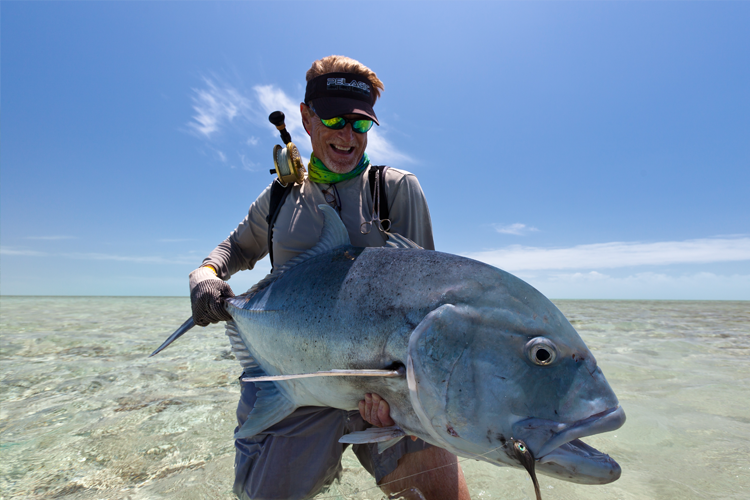In this bright and clear photo, a smiling man stands knee-deep in shimmering, shallow, and crystal-clear water, holding an enormous blue-gray fish, likely a catfish, that's almost as long as he is tall. The man is dressed in a baseball cap, sunglasses reflecting the serene surroundings, a white or grey long-sleeve shirt, and grey pants, with scuba gear visible on his back. His gloved right hand firmly grips the fish's tail, while his left arm supports its hefty body. The massive fish, with its mouth slightly agape, has noticeable fins and a fishing hook with a lure still attached to its mouth, trailing a line off the edge of the image. Behind the man, the sky stretches out in a clear blue expanse with minimal clouds, and the transparent water reveals the light tan sand beneath. The overall atmosphere suggests a moment captured earlier in the day, under the bright midday sun.